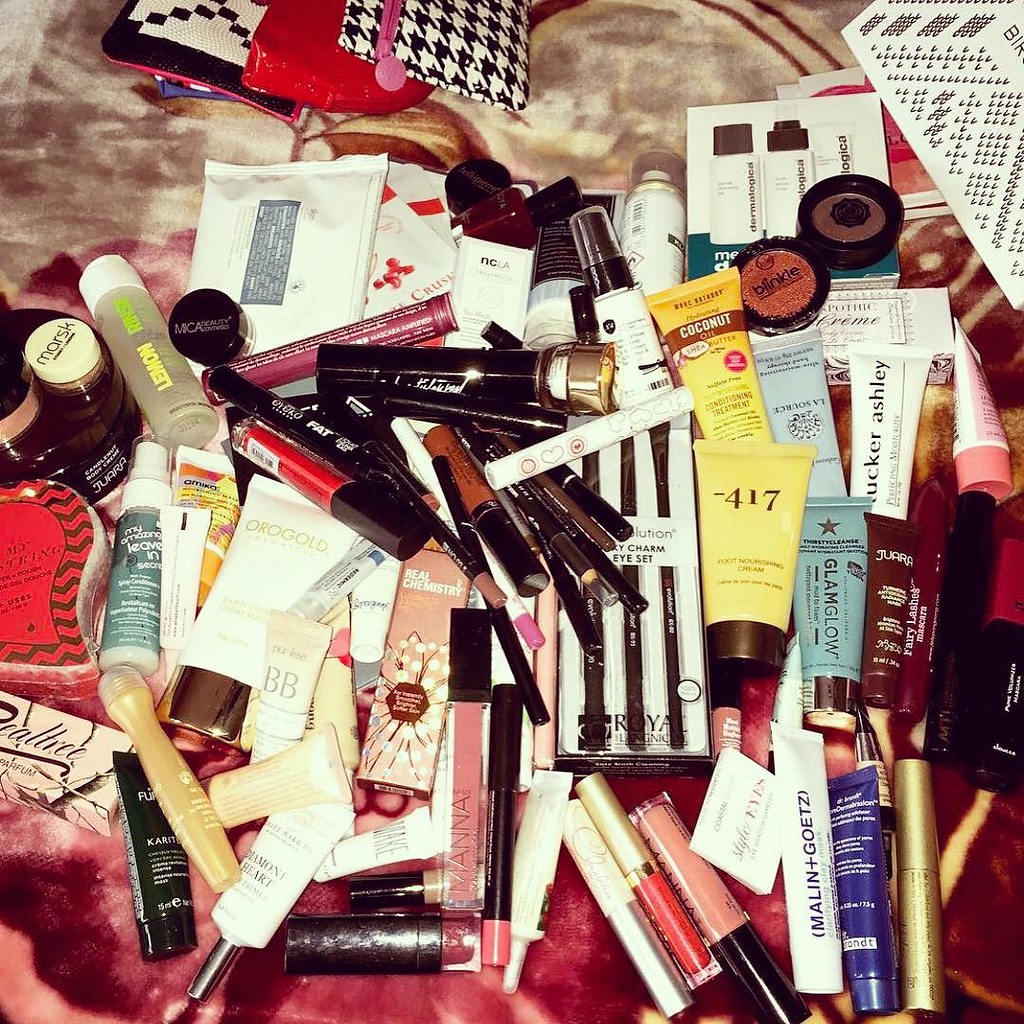This overhead photograph showcases an extensive assortment of travel-size beauty products meticulously arranged on a surface covered with blankets. The collection features approximately 50 to 100 items, encompassing a diverse array of makeup, skincare, and hair care products from various brands. Visible in the assortment are blushes, eyeliners, makeup brushes, lipsticks, lip glosses, creams, and lotions. Each item varies in size, adding to the eclectic feel of the display. The products are evenly spread out across the blanket, creating an impression of abundance and variety. The top-down perspective captures the full extent of the collection in a visually appealing manner.